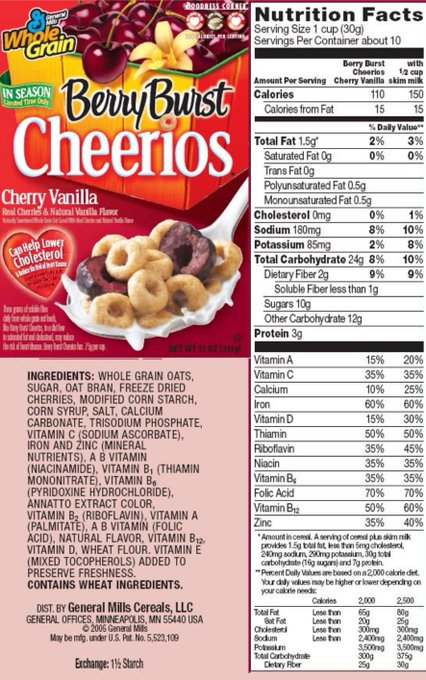The image showcases the back panel of a flattened Berry Burst Cheerios cereal box, meticulously laid out to display both the front and side panels in a contiguous manner. Dominating the upper left-hand corner is the front of the box, vividly illustrated with the text "Berry Burst Cheerios" in bold. A spoon filled with Cheerios and small cherry bits extends from the right side, emphasizing the "Cherry Vanilla" flavor. Accompanying the image, text highlights the inclusion of "Real cherries and natural vanilla flavor." The box's dominant red hue is accentuated with touches of yellow.

Beneath the flavor description, within a heart-shaped emblem adorned with white lettering, it is proclaimed that the cereal "Can help lower cholesterol." Adjacent to this vibrant box front, the right segment of the image reveals the Nutrition Facts panel in detail. This section informs the consumer that a serving size is 1 cup, with the box containing approximately 10 servings. It states that each serving, sans milk, contains 110 calories, increasing to 150 calories when combined with half a cup of milk.